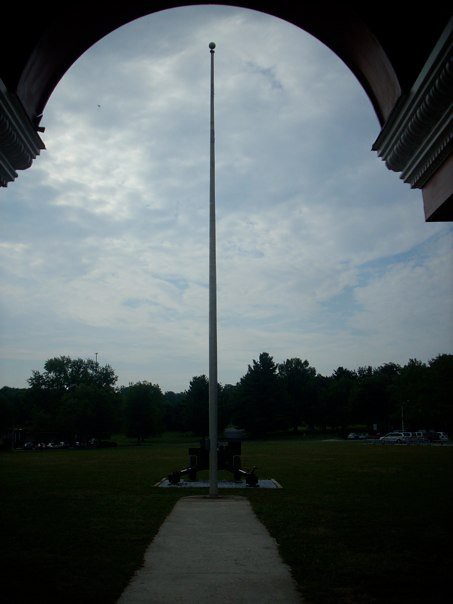This image captures an outdoor scene dominated by a tall, thin pole—likely a flagpole or light pole—with a ball at its top, reaching around 30 feet high. The image is quite dark, lacking contrast, which makes the finer details hard to discern. In the foreground, a concrete sidewalk or dirt pathway leads the eye directly to the pole, bisecting a grassy field. The scene is framed by a large architectural archway from the perspective of the photographer, suggesting they are standing inside or adjacent to a building structure. Further back, multiple cars are parked in a lot, and the area is lined with numerous trees. The sky above is mostly cloudy with intermittent patches of blue, adding a somber tone to the overall composition, which might suggest a setting like a cemetery. The central focus remains on the stark, barren pole set against the predominantly grey sky.